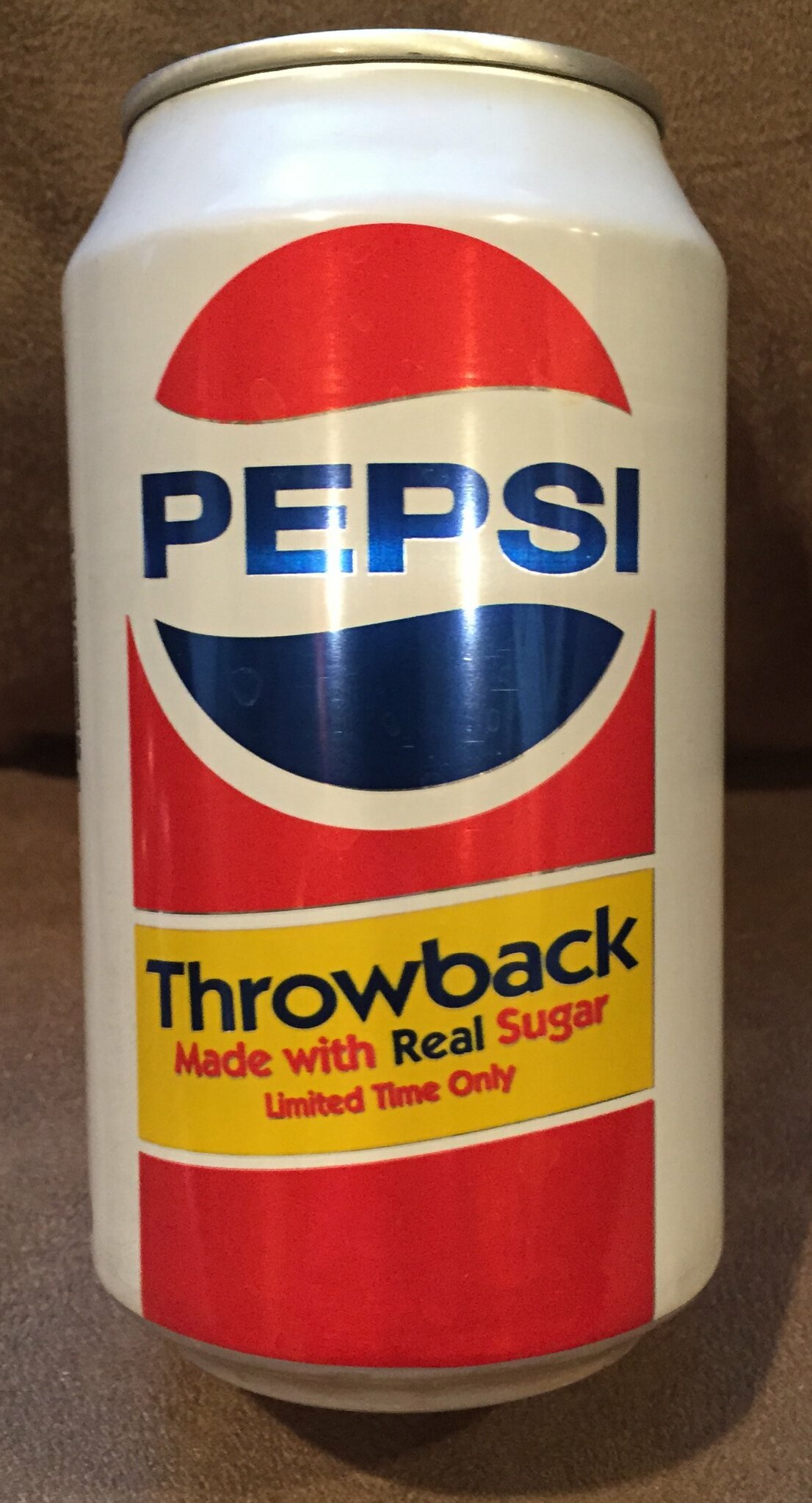This is a detailed photograph of a Pepsi "Throwback" can taken with a regular camera, featuring a retro-style design. The predominantly white can showcases an old-fashioned Pepsi logo. The logo comprises a red swoosh at the top and a metallic blue swoosh at the bottom, forming a circle intersected by a wavy white space with the word "PEPSI" in large blue capital letters. The middle of the can features a yellow banner with the text "Throwback," "Made with real sugar," and "Limited time only" in black and red lettering. Additionally, a red, rectangle-like area with a dome top encompasses the centered text. The entire can is topped with a gray rim, and the background of the image is a brownish-beige color.